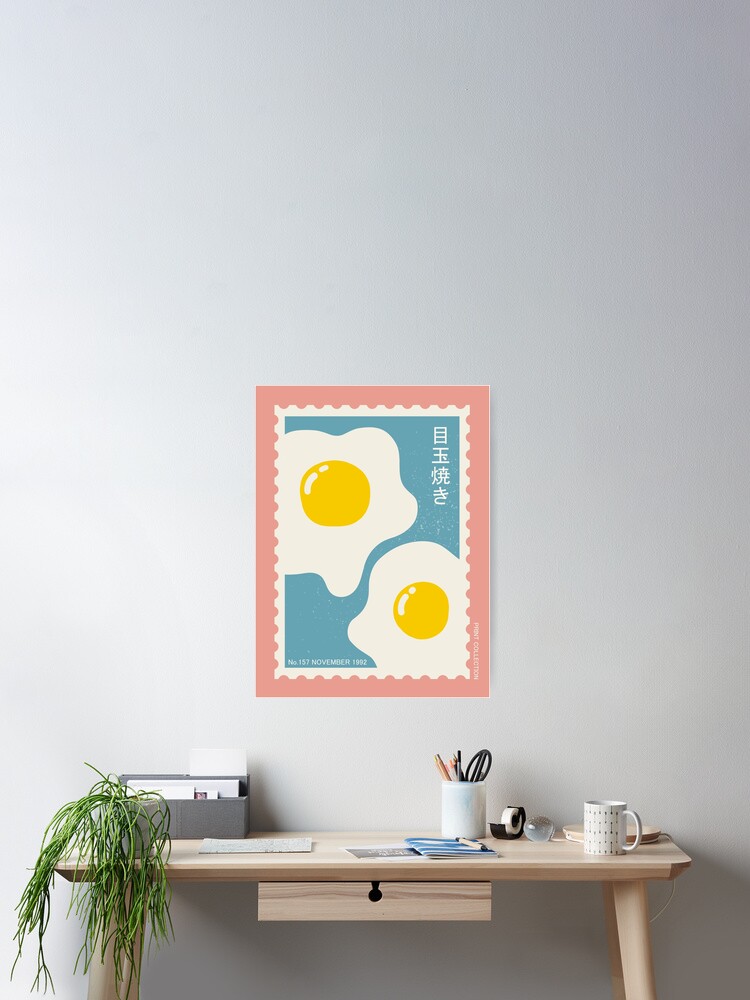In front of a blank white wall, there is a sleek, modern-style wooden desk with a small pull-out drawer in the center. The drawer is a few inches tall and about a foot wide. Atop the desk sits a green, willow-like plant with very long branches. Behind the plant, there's a basket of letters containing various papers, some of which are blue. A cup holding pencils and scissors, a black tape dispenser, a paperweight, a white mug with black designs, and a tall, white table lamp that bends at the halfway point to angle over the desk populate the workspace. On the wall above the desk hangs a picture designed like a postage stamp, featuring two sunny-side-up eggs with visible yellow yolks on a blue backdrop and a pink border. There are also Chinese characters on the stamp-like image. The overall setup is minimalistic, giving the impression of a simple yet functional office space.